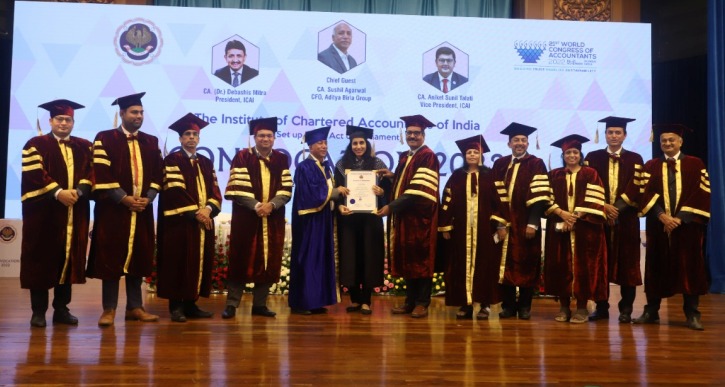This detailed photograph captures a graduation ceremony on a polished, wooden stage, where a dozen individuals stand in a line. The graduates are smartly dressed in burgundy caps and gowns adorned with gold stripes. In the center of the group, a woman in a black gown, holding what appears to be her degree or diploma, is being congratulated by a man in a distinctive blue gown. On either side of her, several individuals, including another man in a large red gown with gold stripes, stand proudly. The backdrop features a large white banner with the text "Institute of Chartered Accountants of India" as well as "25th World Congress of Accountants." The poster also displays images of key figures from the institute. All graduates looking towards the camera share joyful smiles, commemorating this significant achievement.